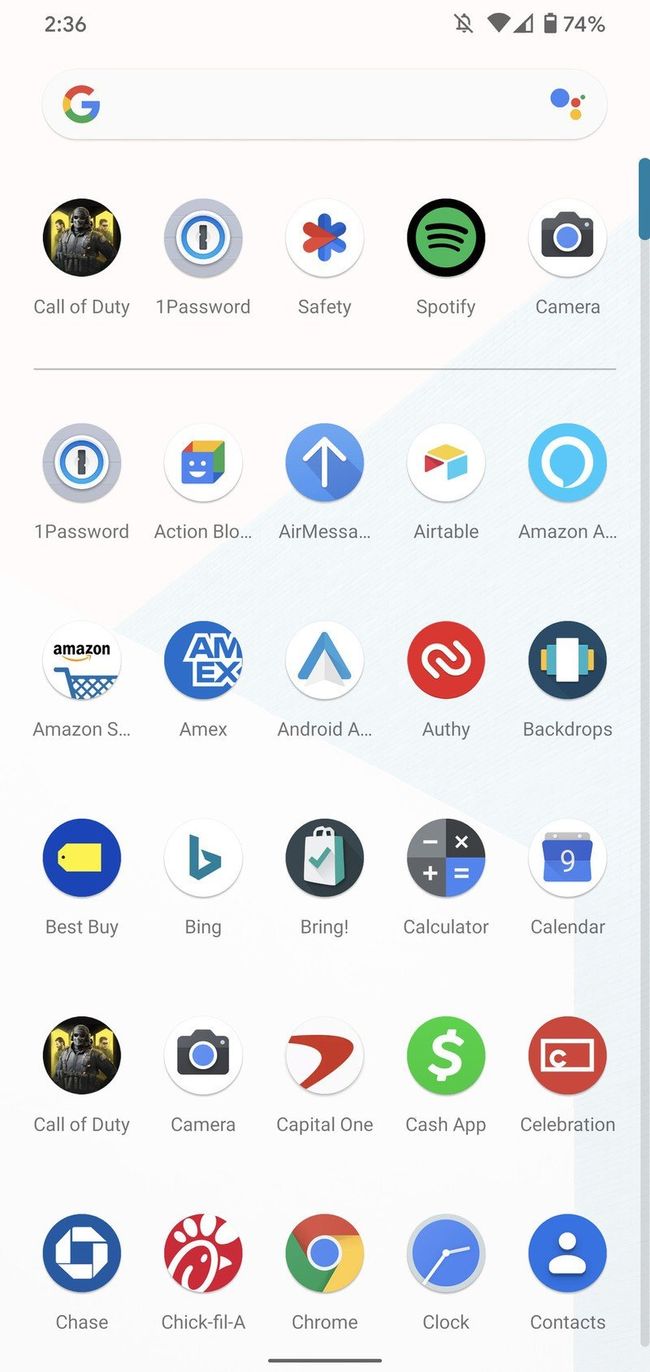The image captures a screenshot of a mobile phone's home screen, taken at 2:36 PM. The phone is set to silent mode, as indicated by a bell icon with a line through it, and it is connected to Wi-Fi with about two out of four bars of signal strength. The battery level is at 74%. Below the status indicators, there is a Google search bar, enabling quick internet searches. The screen displays an extensive array of installed applications, including:

- Call of Duty
- 1Password (appearing twice)
- Safety
- Spotify
- Camera
- Action Blog
- Air Messenger
- Airtable
- Amazon Alexa
- Amazon Shopping
- Amex
- Android
- Authy
- Backdrops
- Best Buy
- Bing
- Bring
- Calculator
- Calendar
- Capital One
- Cash App
- Celebration
- Chase
- Chick-fil-A
- Chrome
- Clock
- Contacts

At the top right corner, a blue scrollbar signifies that there are many more apps available, suggesting a well-populated app library on the device. This section provides a comprehensive view of all the user's installed applications, allowing for easy navigation and access.